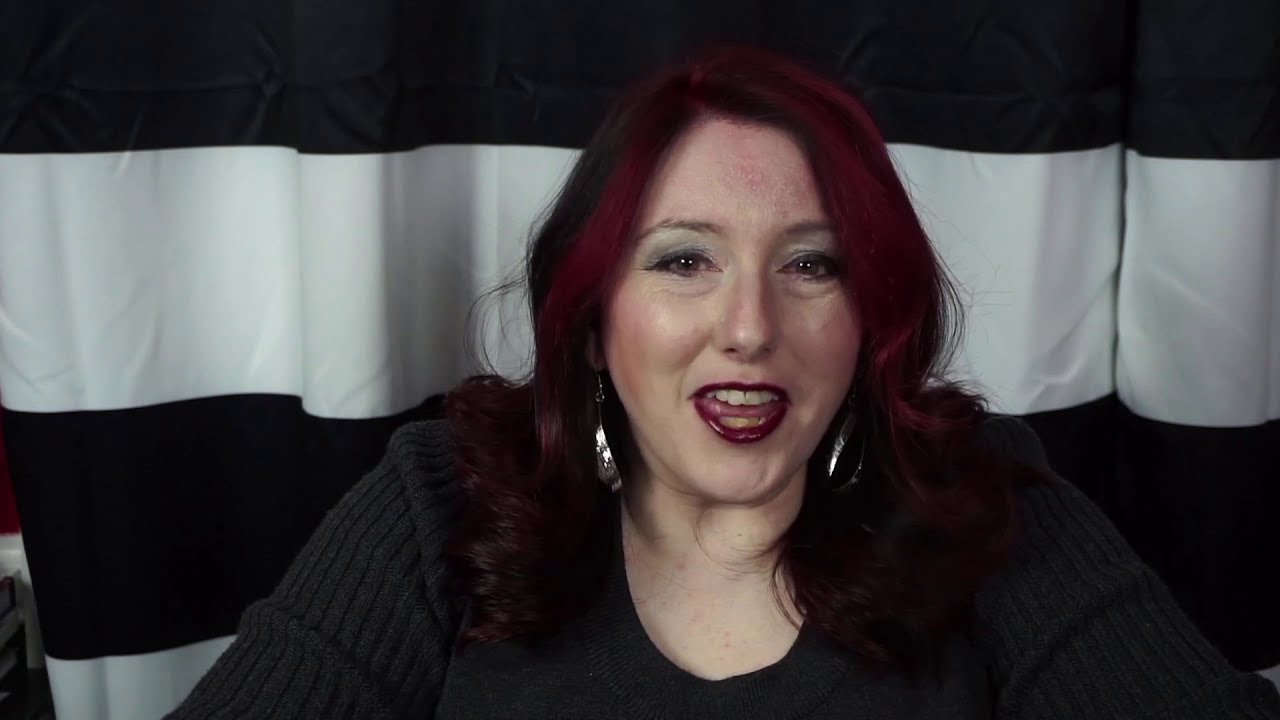This is a detailed color photograph of a woman, slightly off-center and facing the camera, captured mid-speech with her mouth slightly open, resembling a smile. Her hair, originally dark brownish-black, has been dyed burgundy with red streaks towards the front and sides. Her hair cascades down slightly past her shoulders. She has light skin, dark brown eyes, and is wearing ample makeup, including gray eyeshadow, mascara, brown eyebrows, some blush, and deep red lipstick. She is adorned with large silver hoop earrings. The woman is dressed in a long-sleeved black ribbed sweater. She is seated in front of a black and white horizontally striped curtain, with an additional segment of darker red, white, and gray visible in the lower left background. The photograph, measuring approximately seven inches wide by five inches tall, is text-free. Her expression, with an open mouth, suggests that she is speaking about something that brings her joy.